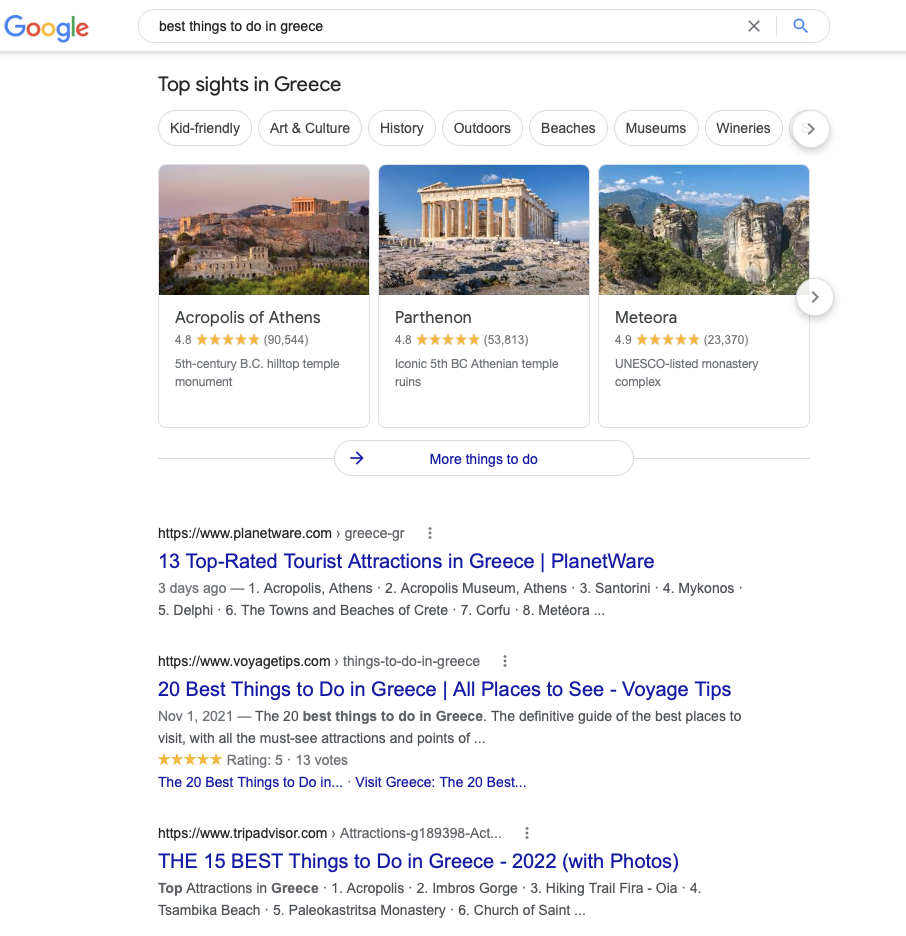This image captures a Google search page for "best things to do in Greece." At the top, the search bar displays the query, while below it, several categories are listed: "Top insights in Greece," "kid friendly," "art and culture," "history," "outdoors," "beaches," "museums," and "wineries." The page highlights three popular destinations:

1. **Acropolis of Athens**: This entry includes a 5-star rating and describes it as a "15th century BC hilltop temple monument." The accompanying image shows the iconic structure perched atop a hill, showcasing its ancient architectural marvels.
   
2. **Parthenon**: Also rated 5 stars, this option is described as the "iconic 5th BC Athenian temple ruins." The image features the well-known remnants of the temple, famous for its historical and cultural significance.
   
3. **Meteora**: Identified as a "UNESCO-listed monastery complex," this option is accompanied by a photograph of striking rock formations with monasteries atop them, highlighting its unique and dramatic landscape.

At the bottom of the image, a blue button labeled "more things to do" invites further exploration. Below this button, three websites are listed as additional resources:
   
- **PlanetWare**: Featuring an entry titled "Top Rated Tourist Attractions in Greece," with the site name written in blue.
  
- **Voyage Tips**: Offering a guide titled "20 Best Things to Do in Greece" with "All places to see," also highlighted in blue.
   
- **TripAdvisor**: Listing "The 15 Best Things to Do in Greece 2022" accompanied by photos, with the website's name similarly highlighted in blue.

This well-organized search result provides a comprehensive starting point for anyone planning a trip to Greece, featuring top-rated historical sites and helpful travel guides.